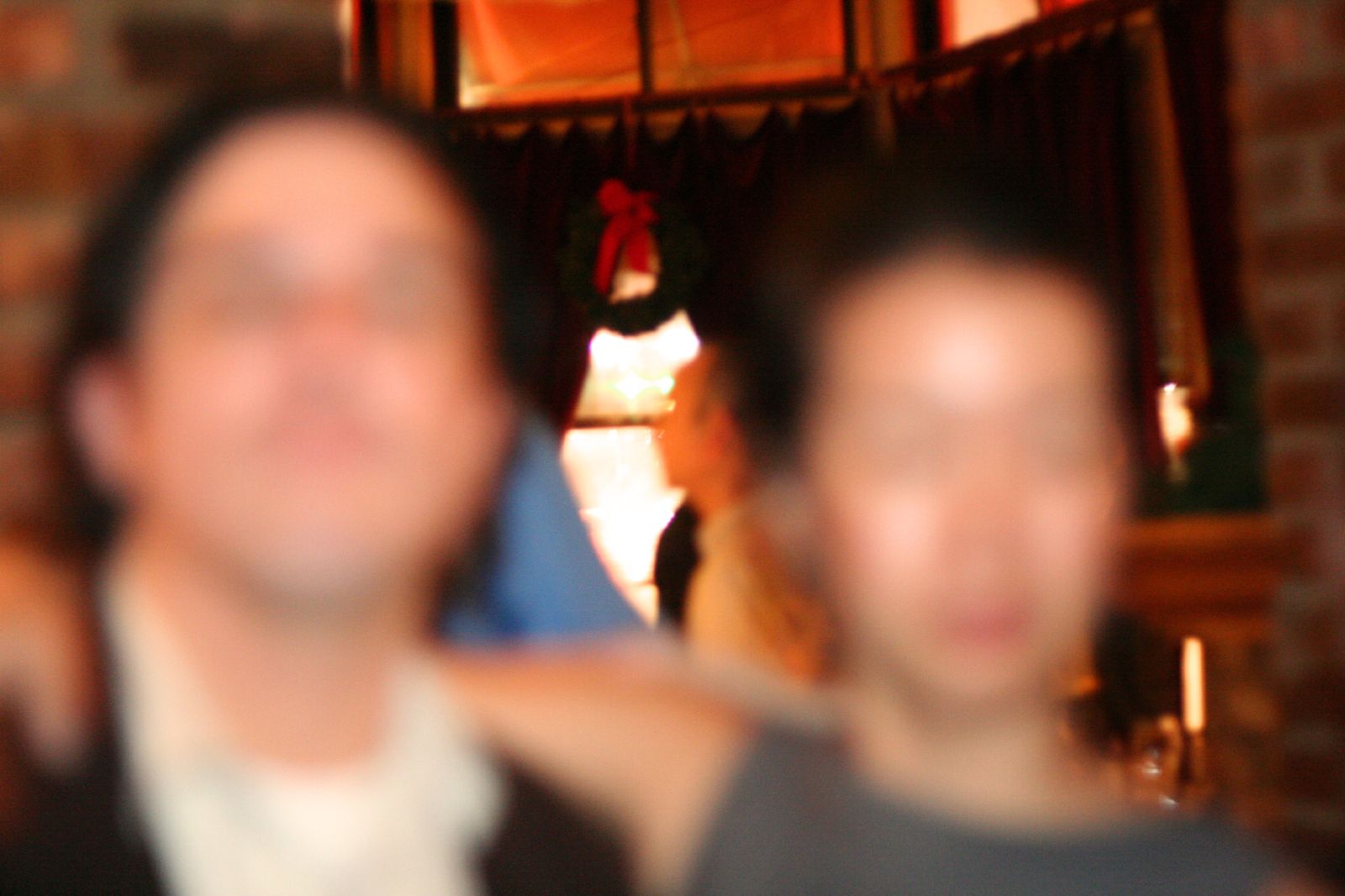This color photograph captures a head-and-shoulders shot of two blurred figures in the foreground, a man on the left and a woman on the right. The man has brown hair that extends slightly past his ears and wears a white shirt underneath a black jacket. The woman, who appears slightly smaller and possibly Asian, has dark hair that seems pulled back and wears a sleeveless gray top with a round collar. Her right arm is wrapped around the man's shoulders, suggesting a close relationship as they both look directly at the camera. Despite the blurriness, certain details emerge in the background. A window framed by dark curtains is visible, with a triangular sliver of sunlight piercing through an opening. Above the man near the window, a green Christmas wreath adorned with a red bow hangs prominently, adding a festive flair. There is also a slightly clearer bricked area on either side of the window, and a candle that appears to be reflected in a mirror above the scene, giving more context to the likely indoor setting.